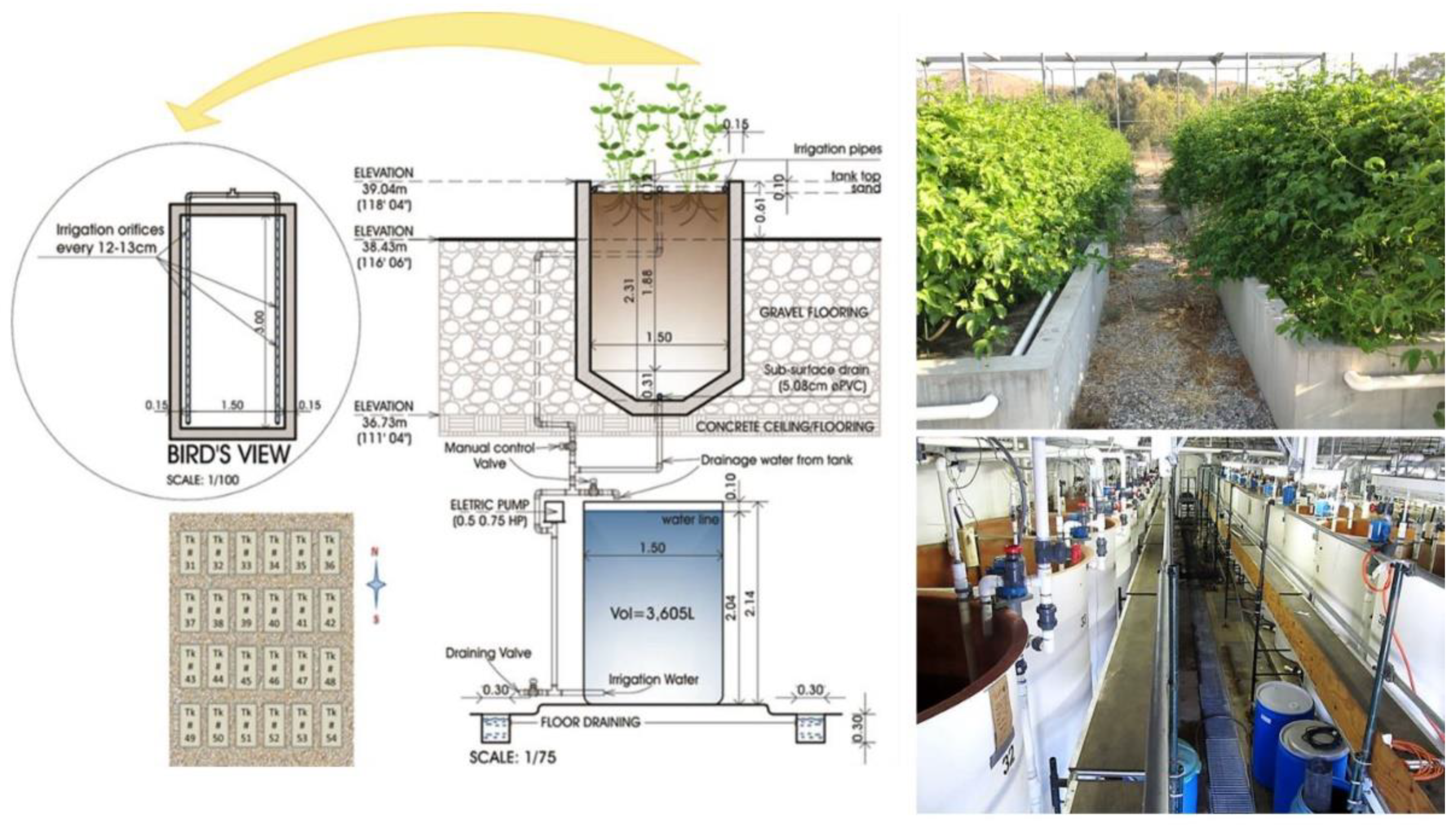This composite image presents a detailed vision for an industrial-style garden design. On the left side, there is a comprehensive architectural diagram illustrating the garden's layout, including elevation details, measurements, and specific areas designated for various plant boxes. The plan highlights a gravel flooring with built-in drainage systems. To the right of the diagram, the top photograph features lush green vegetation housed in large, concrete rectangular garden beds, separated by gravel pathways. Below this, the bottom photograph depicts an industrial factory setting with multiple tanks and vats connected by a network of pipes, likely representing the irrigation system that will manage the garden's water supply. The image captures the seamless blend of careful planning, vibrant planting, and industrial infrastructure.